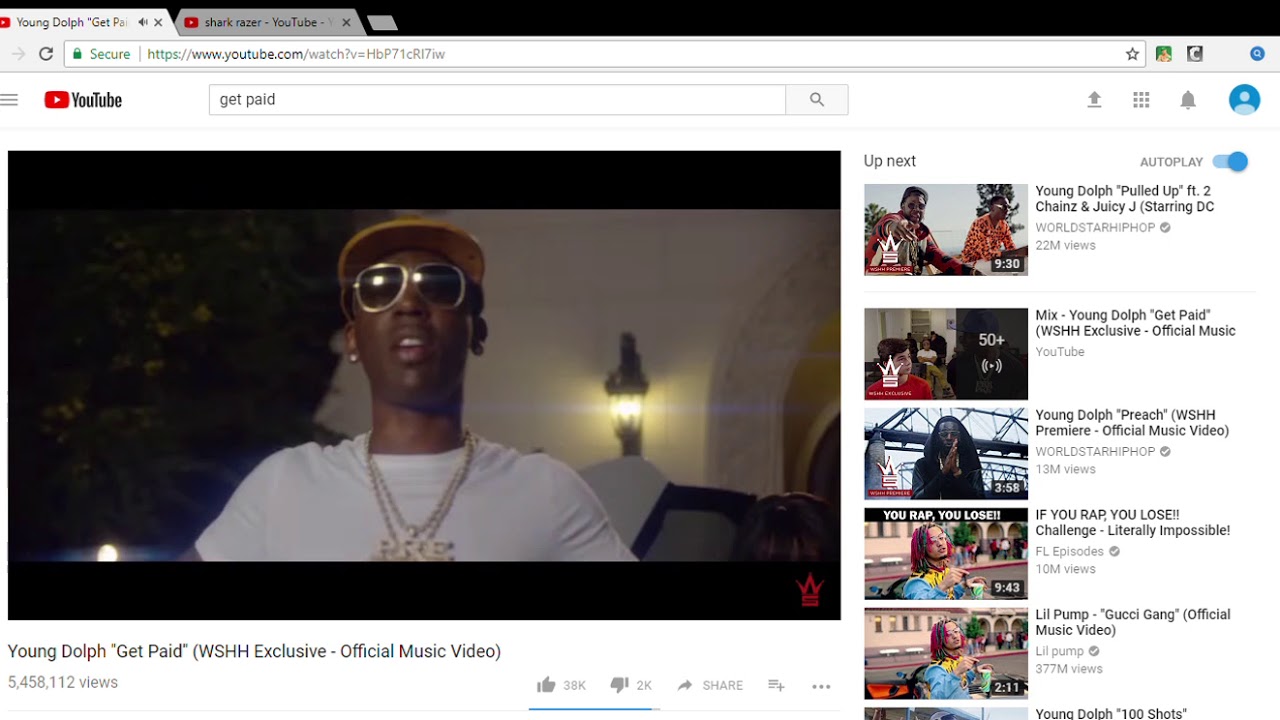A still image from YouTube displays the interface of a music video titled "Young Dolph - Get Paid (WSHH Exclusive - Official Music Video)," which has accumulated 5,458,112 views. The main video shows a young black man, Young Dolph, adorned with a "PRE" chain and wearing sunglasses, a yellow hat, and a white t-shirt. Along the right-hand sidebar, there is a list of suggested videos, including "Young Dolph - Pulled Up (feat. 2 Chainz and Juicy J)," "Mix - Young Dolph Get Paid," "Young Dolph - Preach (WSHH Premiere - Official Music Video)," "If You Rap You Lose Challenge Literally Impossible," and "Lil Pump - Gucci Gang (Official Music Video)."

In the upper left corner, the browser has two open tabs: one labeled "Young Dolph Get Paid" and the other "Shark Razor YouTube," set against a black background. The URL bar shows "www.youtube.com/watch?v=HBP71CR17IW," accompanied by a forward arrow and a refresh icon. On the right side of the toolbar, several extensions are visible along with three horizontal gray lines for options.

The YouTube interface includes the classic red play button and "YouTube" text in black on the left. In the search bar, the query "Get Paid" is visible. Additionally, the interface features various icons on the right, including download, grid style, notification, and profile icons.